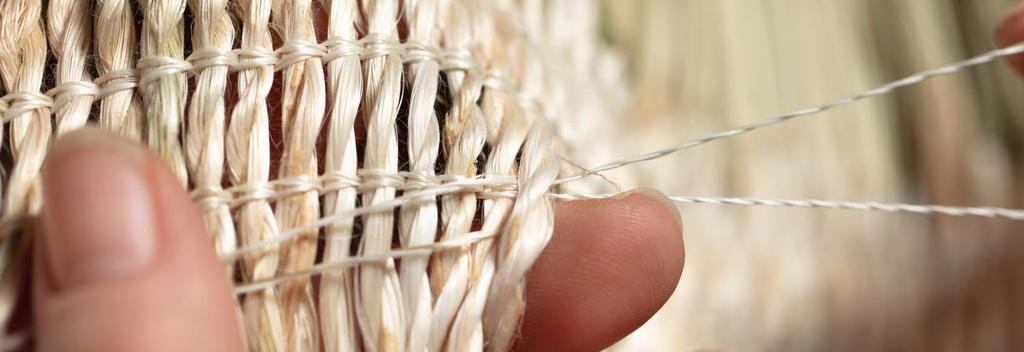In the photograph, a woman's two fingers—her thumb on the left and her index finger in the center—are intricately working on weaving a basket or a jute structure. The crafting process involves stitching a white thread through vertically positioned, light beige strands, forming a knot-like pattern. This close-up shot emphasizes the tension in the thread pulled taut to the right. The shallow depth of field highlights the focus on the thumb and weaving action, while the background appears blurred with streaks of beige, giving the impression of an elongated, intricate woven object. The image intricately captures the delicate and detailed craftsmanship involved in the weaving process.